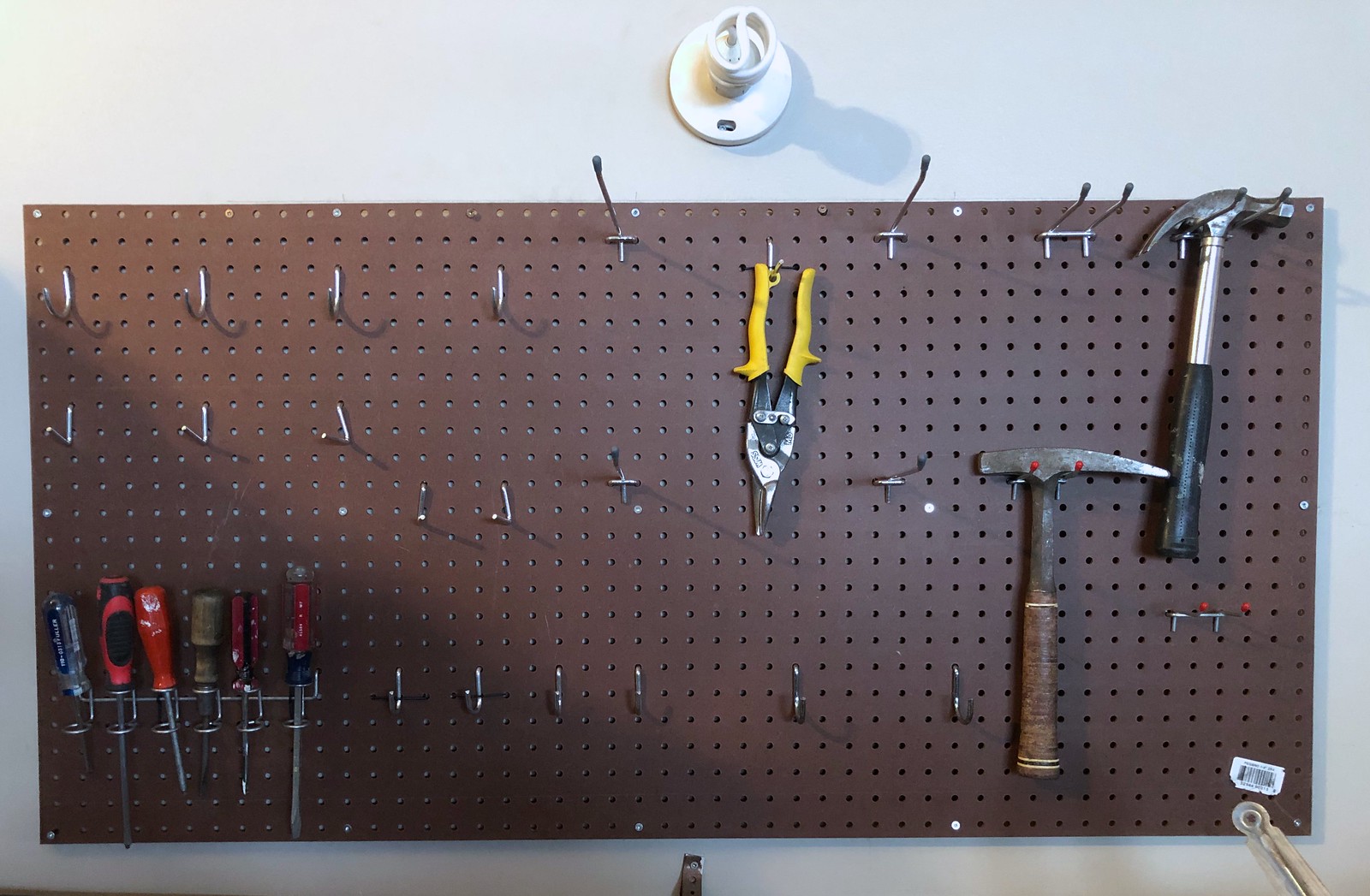This detailed photograph captures a landscape-oriented view of a large brown pegboard mounted on a white wall. Above the pegboard, centrally placed, is an unlit LED light fixture. The pegboard itself is robustly attached to the wall and organized with approximately 30 hooks of various types, including L hooks, S hooks, and longer bracket hooks.

On the pegboard, starting from the top right-hand corner, there is a hammer with a black handle secured by two brackets. Adjacent to this hammer is another hammer with a brown handle. Slightly to the left, more centrally positioned at the top, hangs a pair of pliers with yellow handles. Beneath these pliers is another tool with a brown handle, possibly for cutting.

On the bottom left-hand side of the pegboard, there is an organized rack holding six screwdrivers with handles pointing downward. From left to right, the colors of the screwdriver handles are blue-silver, red-black, red-coppery, red with a black stripe, and red with a black top. The arrangement of tools and the meticulous use of hooks and brackets indicate a well-organized workspace.